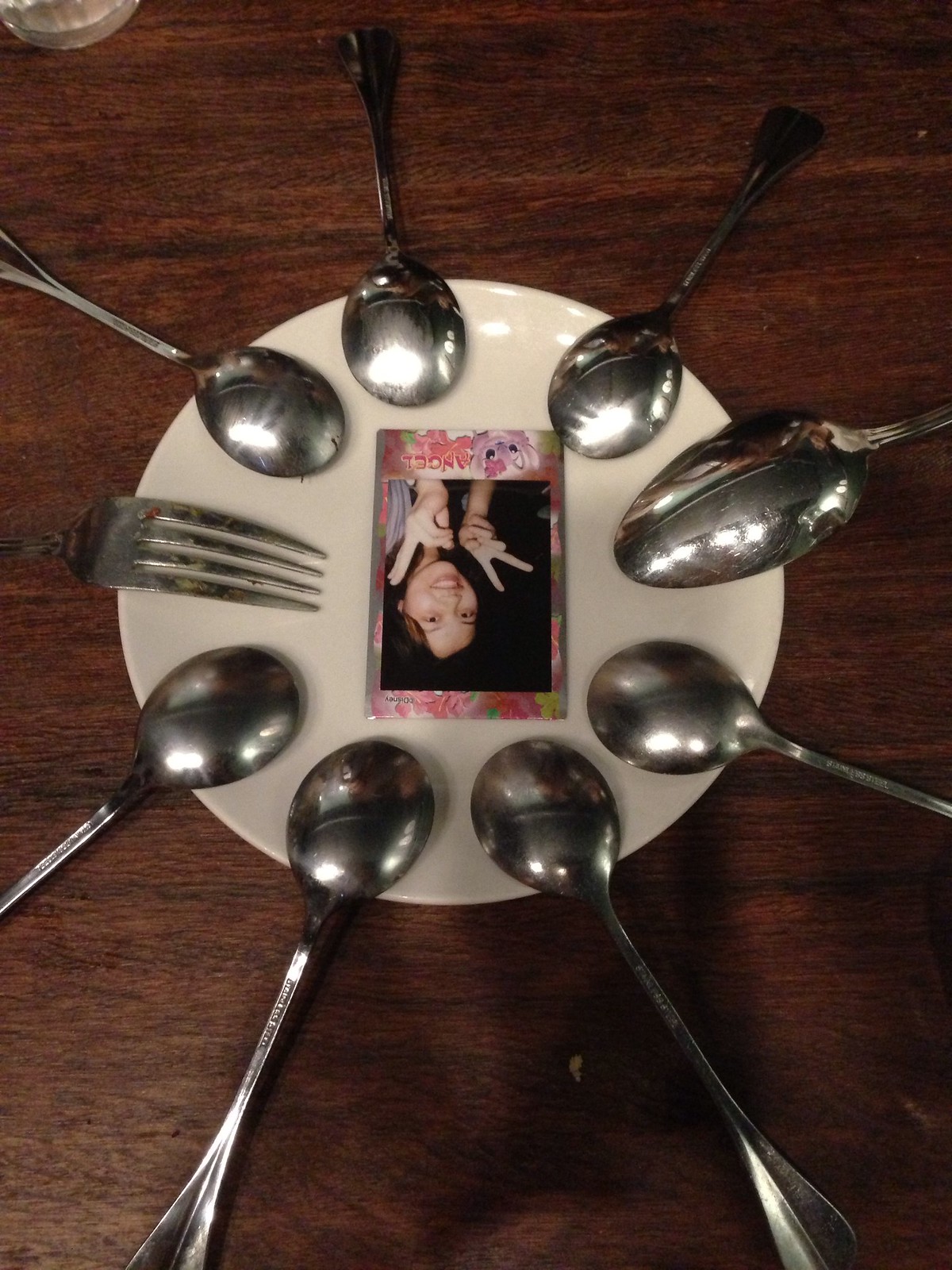The image is a detailed photograph from a top-down perspective showcasing a brown wooden table, possibly made of either real wood or Formica. Centered on the table is a round, white plate. Positioned in the middle of the plate is a photo card bordered with pink and floral multicolored designs. The photo on the card depicts a young woman, likely Asian with long dark hair, flashing the peace sign with both hands, though the image is upside down in the orientation of the photograph. Encircling the plate are eight pieces of silver-colored silverware arranged face down like the petals of a flower, with the bowls of four soup spoons radiating from the bottom arc of the plate, three more spoons (possibly soup or teaspoons) arrayed around the top, and a large serving spoon on the right. Additionally, there is a single fork placed on the left side of the plate. The upper right corner of the table also partially shows the base of a small vase or a similar object.